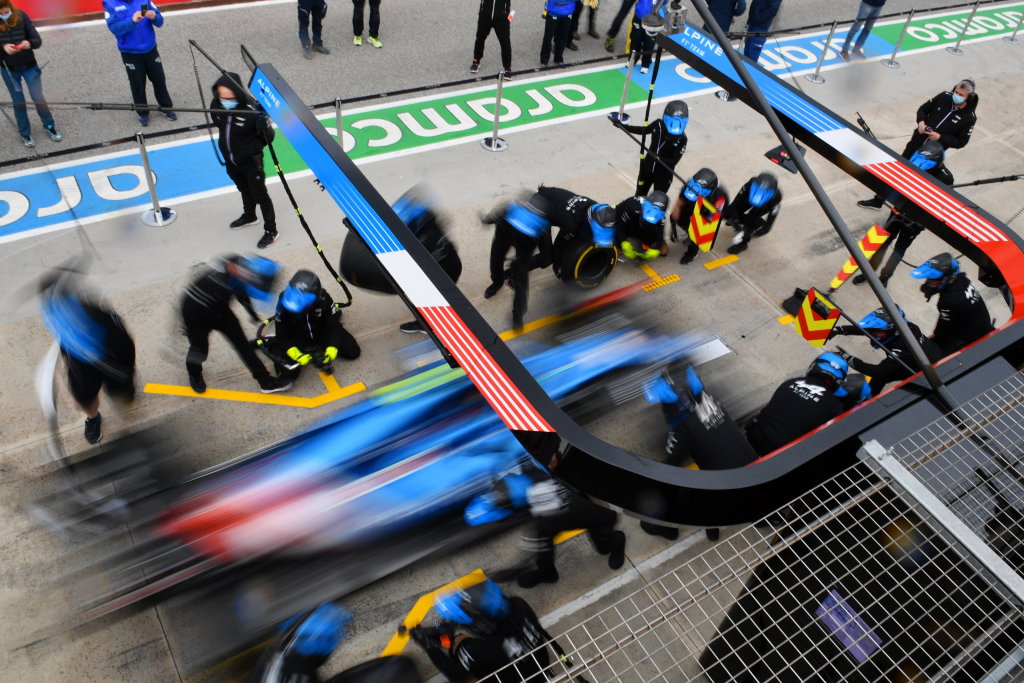The image captures a dynamic moment at a pit stop during a high-speed racing event, likely a Formula One race. The photograph is taken from an overhead perspective and utilizes a slow shutter speed, causing the moving race car and pit crew to appear heavily blurred, while the static elements like the tarmac ground remain in sharp focus. The race car, adorned in blue, red, and black, is captured in motion post-pit stop, sitting on grey asphalt marked with yellow, green, and blue lines. The pit crew, dressed in matching blue, white, and red uniforms, are poised and ready, some already moving to change tires and refuel the car. Above the scene, there is a black metal overhang featuring blue, white, and red stripes. Background details include other team members and possibly family members standing behind a cordoned-off section, as well as a section of the pit lane marked with the team's name, which appears upside down and unreadable in the photograph.